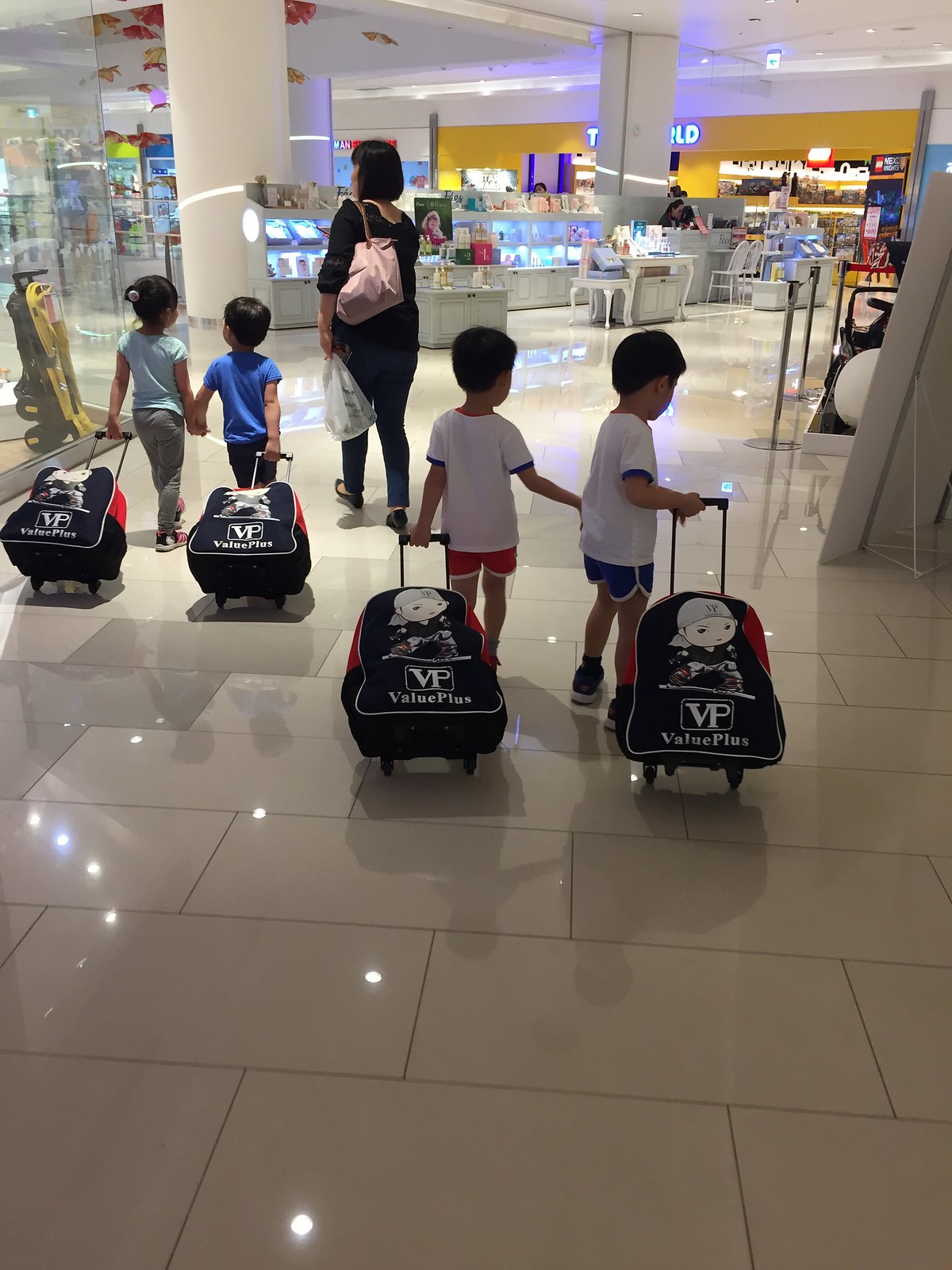In this photograph, a woman, likely a mother, is seen walking through an expansive, modern airport with four children. The floor is adorned with large, glossy white rectangular tiles that reflect the abundant lighting throughout the space. The woman, dressed in a black shirt and blue jeans, carries a plastic bag in her left hand and a pink purse slung over her shoulder. She has black hair. 

The four children are divided into two groups. In the front group, a boy in a blue shirt walks alongside a girl in a green shirt. Behind them, two boys wear matching white t-shirts, one paired with red pants and the other with blue. Each child pulls a similarly designed piece of luggage — navy blue with a red front displaying a "Value Plus" (VP) logo and an anime-style character.

The backdrop features a brightly lit storefront, showcasing various colorful merchandise on illuminated shelves, giving the entire scene a vibrant and bustling atmosphere. The store has an open entrance without a door, seamlessly extending from the shiny tiled floor of the airport.